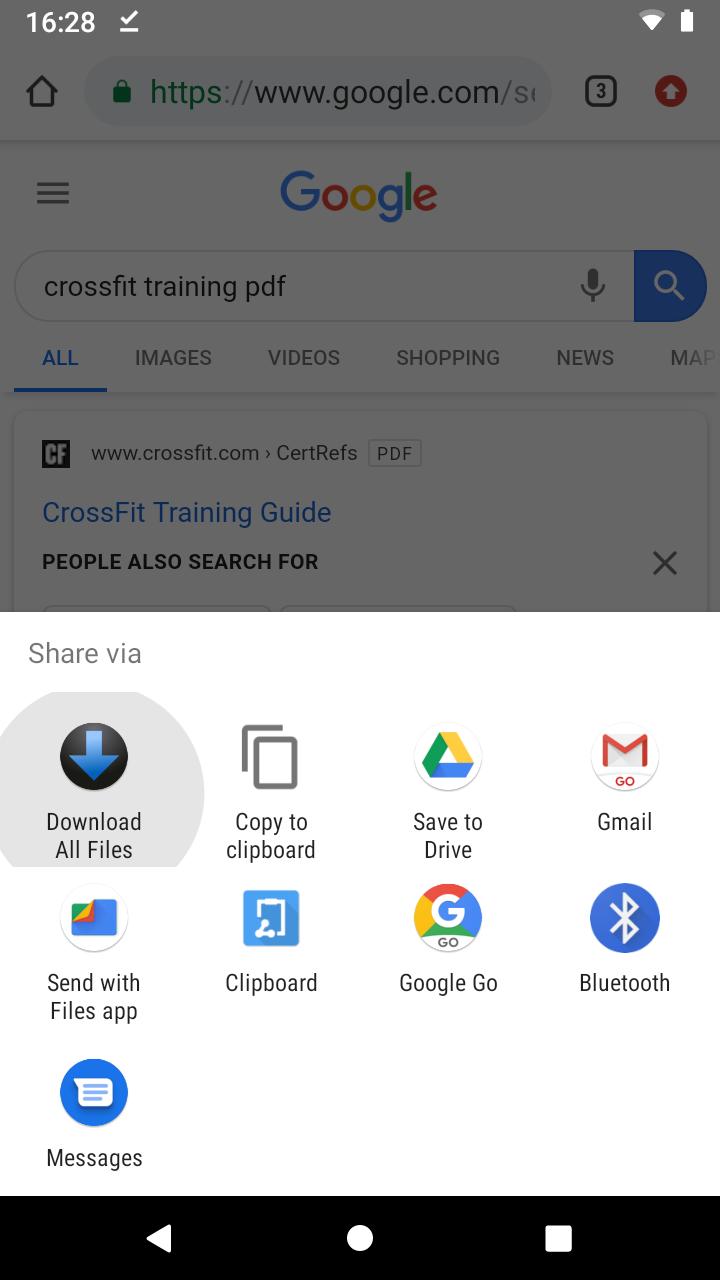This image is a screenshot of a smartphone display, divided into two primary sections. The upper half shows a Google search results page, where the search query entered is "CrossFit Training PDF." The prominent Google logo sits atop the page, followed by a search bar containing the query. The first result is a link to a CrossFit training guide, provided by CrossFit.com, highlighted in blue. Below this link, there is a suggestion section labeled "People also search for," with an 'X' icon for dismissal on the right. The top portion of this section appears to be slightly obscured or blacked out. 

In the lower half of the screen, a share menu is displayed titled "Share Via," presenting nine different options for sharing the content. These are laid out in a grid with four icons in the top row, four in the middle, and one alone in the bottom row. The sharing options include: Download All Files, Copy to Clipboard, Save to Drive, Gmail, Send with Files App, Clipboard, Google Go, Bluetooth, and Messages.